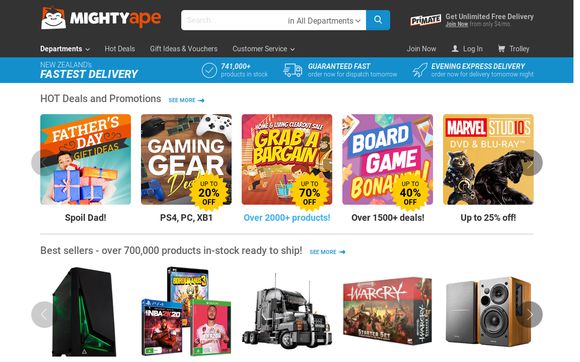In the image, the top part of the background is black with a central graphic. The graphic depicts a white and black figure, possibly a monkey or similar creature, over a red background. To the right of this graphic is a stylized text that reads "MIGHTY" in all capital letters in white, followed by "Ape" in red, lowercase letters. Below this is a search box. Most of the search box's background is white, but the right-hand side is blue featuring a white magnifying glass icon. The left side of the search box has "SEARCH" in very light gray text, followed by "in all departments" in black. Below the search box, "PRIVATE" is written in black, followed by "UNLIMITED FREE DELIVERY" in white, with a prompt to "JOIN NOW."

The next row contains several options: "DEPARTMENTS" in white, followed by "HOT DEALS," "GIFT IDEAS," "VOUCHERS," "CUSTOMER SERVICE," "JOIN NOW," "LOG IN," and "TROLLEY." This row is set against a blue background. Below this, a tagline declares in white text, "NEW ZEALAND'S FASTEST DELIVERY," followed by details of "741,000+ PRODUCTS IN STOCK GUARANTEED." There are prompts to "ORDER NOW FOR DELIVERY TOMORROW" and "EVENING EXPRESS DELIVERY." 

Another section, with a white background and black text, showcases "HOT DEALS AND PROMOTIONS," accompanied by a blue button that says "SEE MORE." Further down, in black text against a white background, it reads "SPOIL YOUR DAD" followed by mentions of "PS4, PC, AX, and B1." In blue text, it states "OVER 2,000+ PRODUCTS." Concluding this part are statements about "OVER 1,500+ DEALS" and "UP TO 25% OFF AS WELL" in black text.